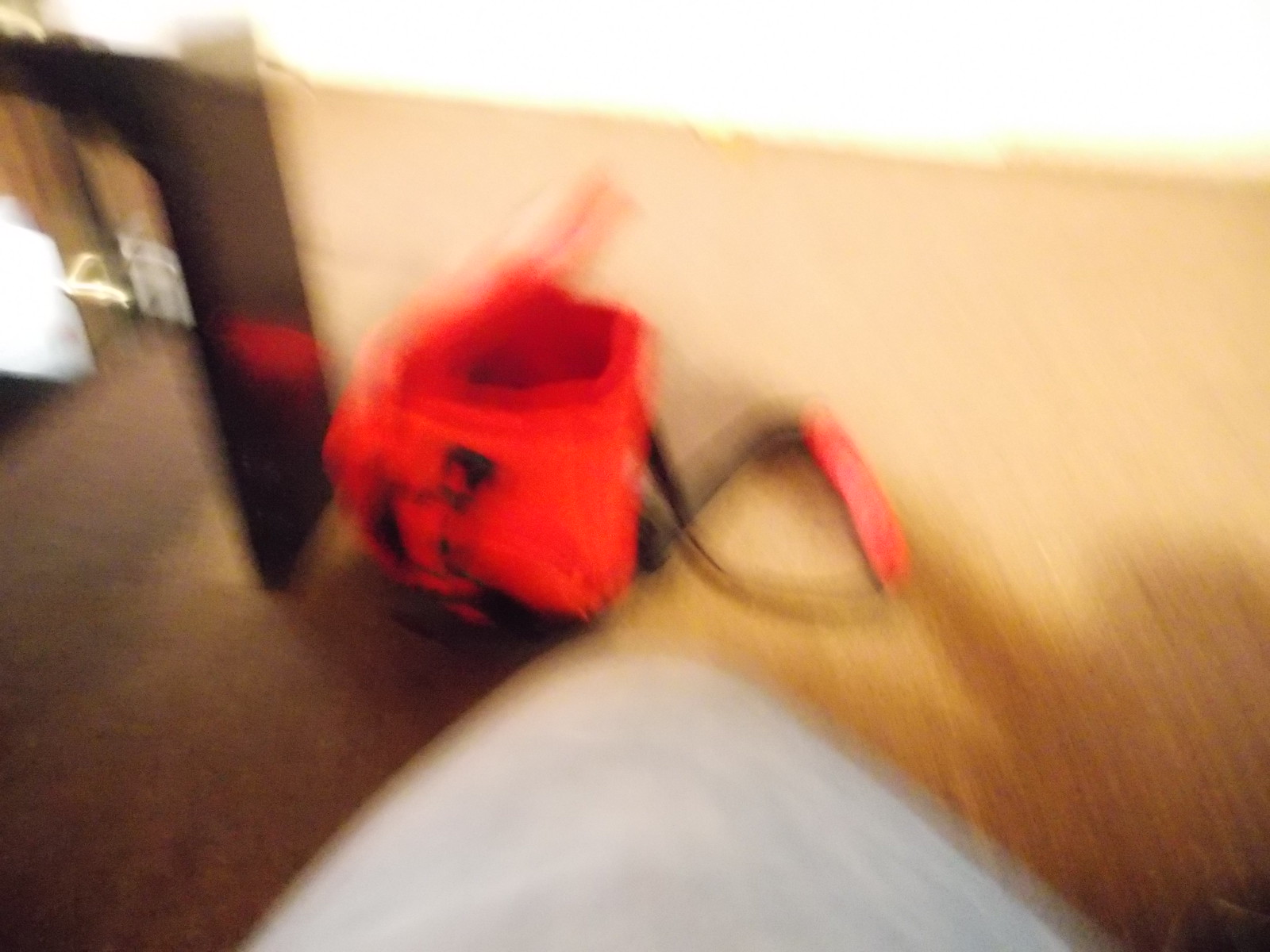The image is an extremely blurry photograph of a room with a brown wall and a dark brown wooden floor. In the center bottom of the image, there is a white, square-shaped object. To its right, a brown item is leaning against the wall, with a red object draped across it. This might be a shop vac due to parts of it appearing black. On the left side of this brown item, there is a red object, possibly a rucksack or bag, featuring black straps. Additionally, in the upper left corner, there's a vertical black bar or wooden frame, possibly framing a doorway, with some light streaming in. The wall to the right of the rucksack is a light cream color. The overall picture is so blurred that identifying precise details is challenging, but the predominant colors and shapes suggest various household items and furniture scattered around.